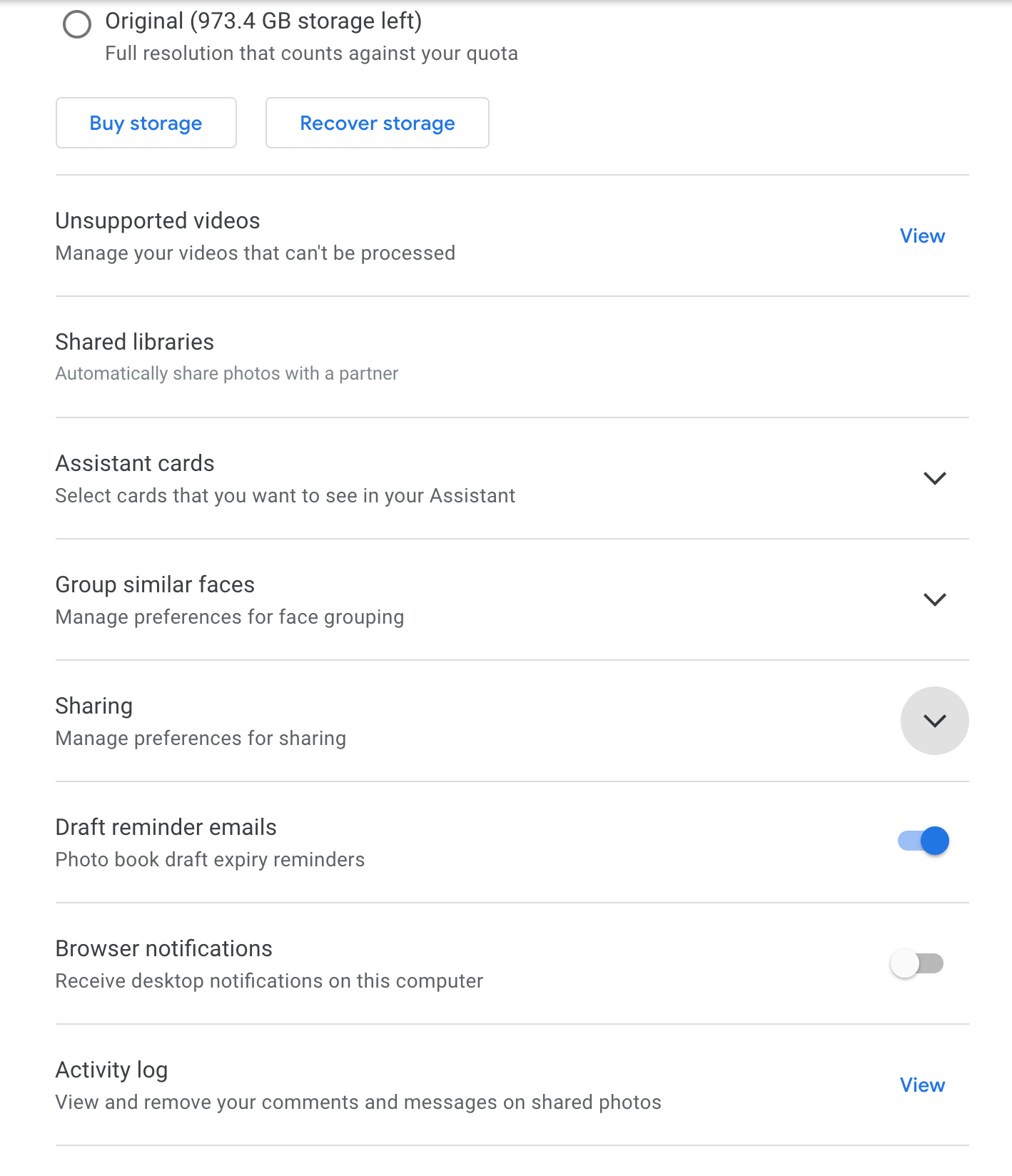Here is the cleaned-up and detailed caption for the image:

---

The image displays a settings menu for Google Cloud Storage. At the top, a gray horizontal bar spans across the screen. Below, there's a black circle accompanied by black text that reads "Original (973.4 GB storage left)". In smaller text underneath, it states "Full resolution that counts against your quota". 

Two white buttons with gray outlines and blue text are located beneath this: the one on the left reads "Buy Storage," and the one on the right says "Recover Storage". Following this section is another gray divider.

Next, in black text, it states "Unsupported Videos," with an option to "Manage videos that can't be processed" next to it in blue text. Another gray divider follows.

Continuing down, a section titled "Shared Libraries" in bold black text appears. Under it, in smaller text, it reads "Automatically share photos with a partner," followed by another divider.

The following section is "Assistant Cards," with a description beneath it saying "Select cards that you want to see in your Assistant" and a black downward-arrow icon to the right. Another divider follows.

The next section is "Group Similar Faces," with a subtext saying "Manage preferences for face grouping" and a black downward-arrow icon beside it, followed by another divider.

The "Sharing" section comes next, with an option to "Manage preferences for sharing" and a gray circle with a black downward-arrow icon on the right.

Underneath another divider is "Draft Reminder Emails," with a description reading "Photo book draft expiry reminders" and a light blue switch indicating it is turned on, with a blue dot on the right side.

Another section, "Browser Notifications," follows, with a description "Receive desktop notifications on this computer." It features a white circle on the left with a gray inactive slider on the right.

At the bottom, the final section is "Activity Log," with instructions to "View and remove your comments and messages on shared photos" and an option to "View" in blue text. Another gray divider follows this section.

---